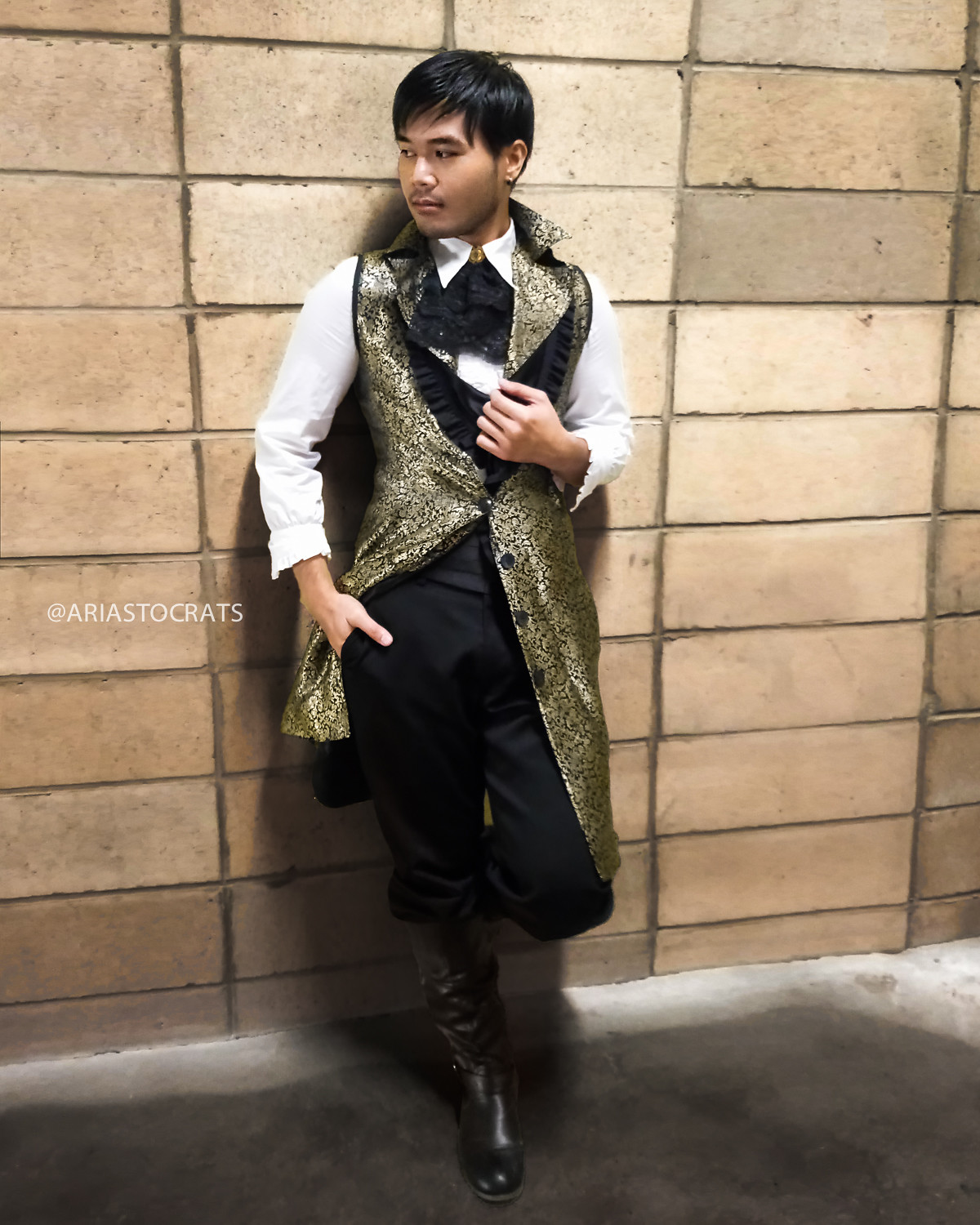This photograph features a young man of likely Asian descent, possibly Filipino. He stands confidently against a white brick wall, roughly textured with bricks that are significantly large, around three feet in length and one foot in height. His attire is notably sophisticated and high-class: he wears black pants paired with black boots, a white shirt underneath a long, gold-embroidered vest-like coat that extends to his knees, adorned with black buttons. One hand rests casually in his pocket while the other grasps the lapel of his coat. Additionally, he has a slight mustache and his short black hair complements his refined appearance. He gazes thoughtfully to his left, exuding an air of confidence though seemingly disengaged, as if lost in thought. Near him is the word "ariastocrats," possibly a reference to his social media handle. The setting, despite his extravagant clothing, appears to be a gritty, urban environment, possibly a subway.